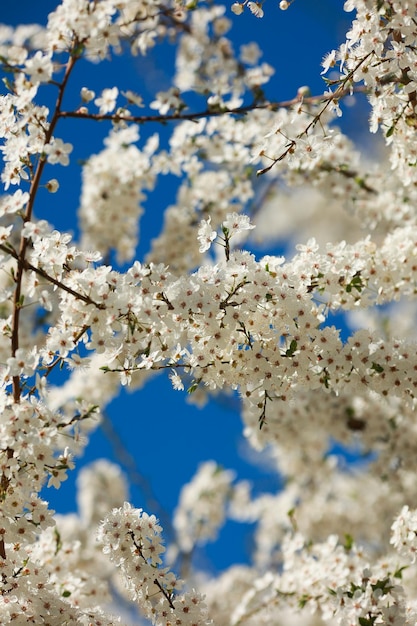A sunny day illuminates an outdoor scene featuring the detailed branches of a flowering tree. Against a backdrop of a vibrant blue sky, the tree's branches are adorned with numerous white flowers, each with four to five petals and a darker center, creating a striking contrast. The thin, brown branches appear almost lost beneath the clusters of delicate blossoms, some of which blur slightly into the background where more flowering treetops can be seen. The light blue sky ensures a clear and bright atmosphere, highlighting the bunched white flowers that dominate the scene.